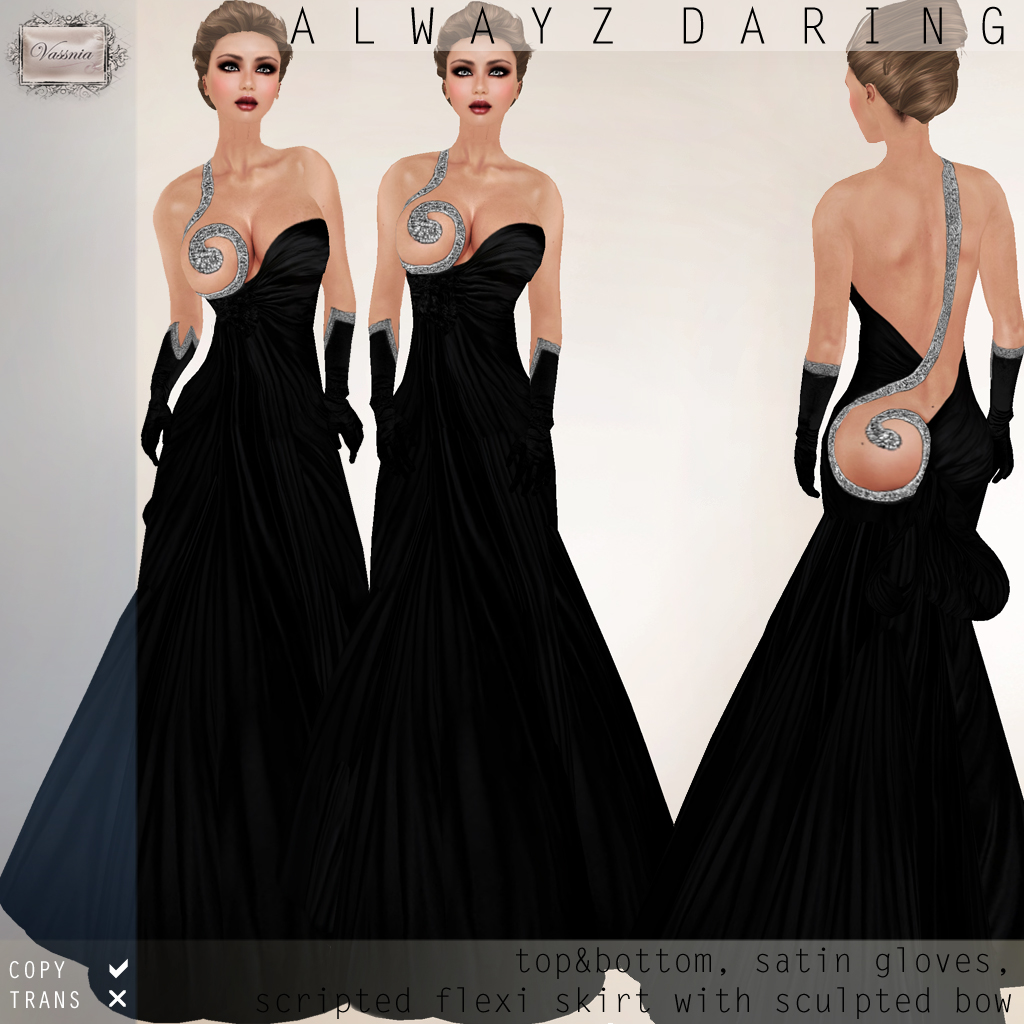This image is a vertical, rectangular computer art advertisement featuring three identical mannequins or robotic-looking women wearing an unusual, elaborate black dress. Each mannequin sports short brown hair and dramatic makeup, including staring eyes and lipstick. The dress is long and black, flaring widely at the bottom. The design uniquely features one shoulder bare, with a single black glove adorning each arm.

On the left side of the image, two mannequins face forward. Their dress covers only the right breast, with the left breast adorned by a distinctive, glittery element, described variously as pink with a blue edge or curly and silver. This piece extends over their shoulder and cascades down to cover part of their back and buttocks.

To the right, the third mannequin stands with her back to the viewer, showcasing the dress's extremely low cut. This rear view reveals the same glittery element, here described as a gold curlicue, which covers part of her back and extends over her shoulder. Her back is fully exposed down to her buttocks, except for the glittery, sculpted piece. All three mannequins wear long black gloves.

At the top of the image, the text "Always Daring" reinforces the bold nature of the attire. Additional promotional content, featuring phrases such as "a top and bottom set in gloves, a scripted flexi skirt with sculpted bow," is inscribed at the bottom, suggesting an avant-garde design focus. The name of the company appears in the lower left corner, embossed on a fancy, presumably silver pillow.